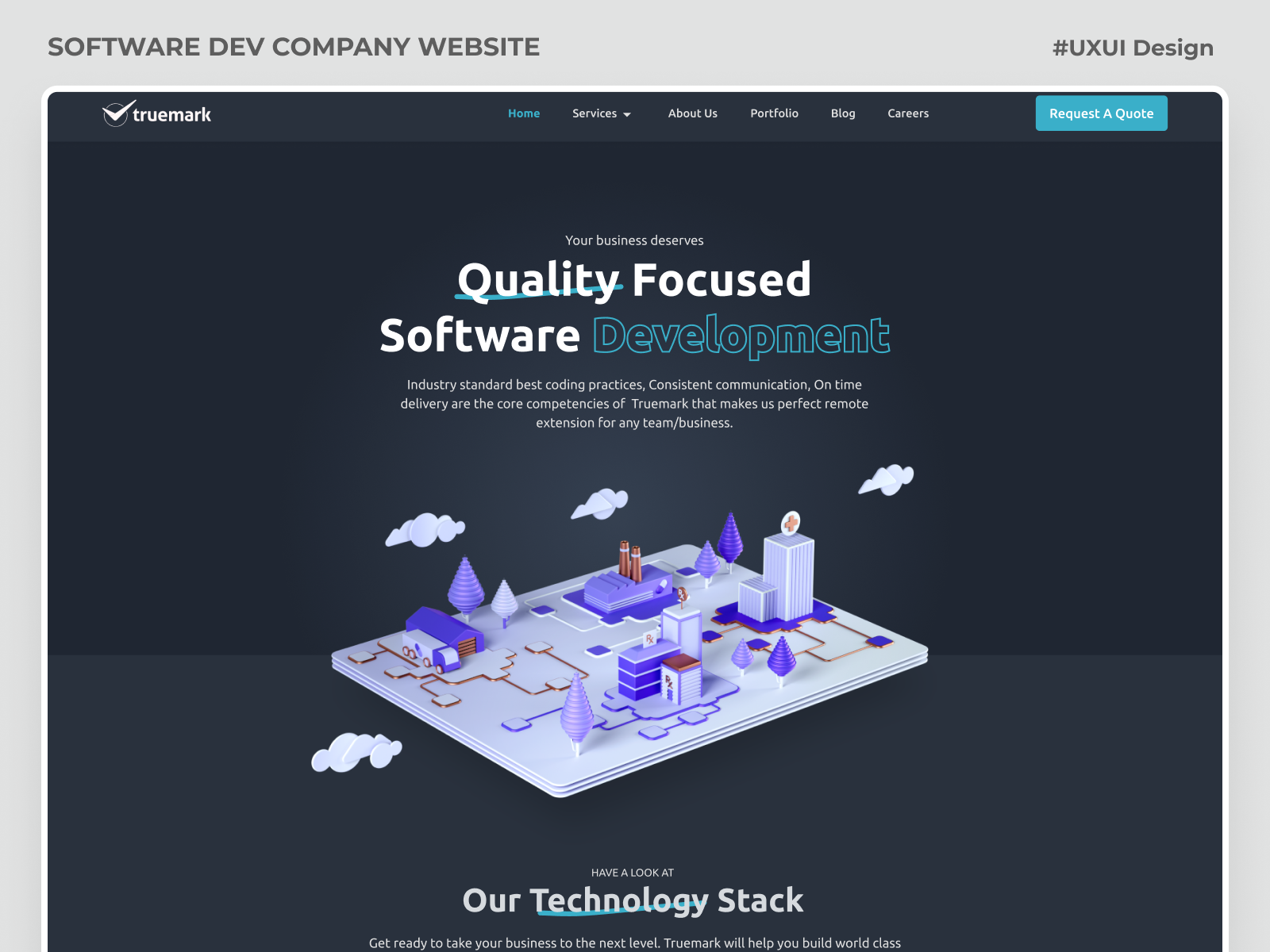The desktop screenshot showcases a web page from a software development company's website. The top left corner features a light gray background with the text "Software Dev Company Website," immediately followed by the hashtag #UXUIDesign. 

A prominent square section with a dark navy background reveals the company name "TrueMark" situated in the top left. The logo resembles a clock displaying 10:10, with the hour and minute hands positioned accordingly. 

To the right of the logo, there are navigation tabs including "Home" (highlighted in blue), "Services" (with a dropdown menu), "About Us," "Portfolio," "Blog," and "Careers." A notable feature is the light blue rectangular "Request a Quote" button.

Beneath this, a headline reads, "Your business deserves quality-focused software development," with "Quality-focused software" in a large white font and "Development" in a slightly smaller light blue font, with semi-transparent letter centers. The next text line highlights TrueMark's competencies such as industry-standard best coding practices, consistent communication, and on-time delivery, positioning the company as an ideal remote extension for any team or business.

The page also features a 3D illustration of a small city with an amusing art style, including four clouds in shades of white and light purple. The cityscape includes a factory with two towering chimneys and a couple of buildings.

At the bottom of this section, the text invites viewers to explore their technology stack with statements like "Have a look at our technology stack" and "Get ready to take your business to the next level. TrueMark will help you build world-class solutions."